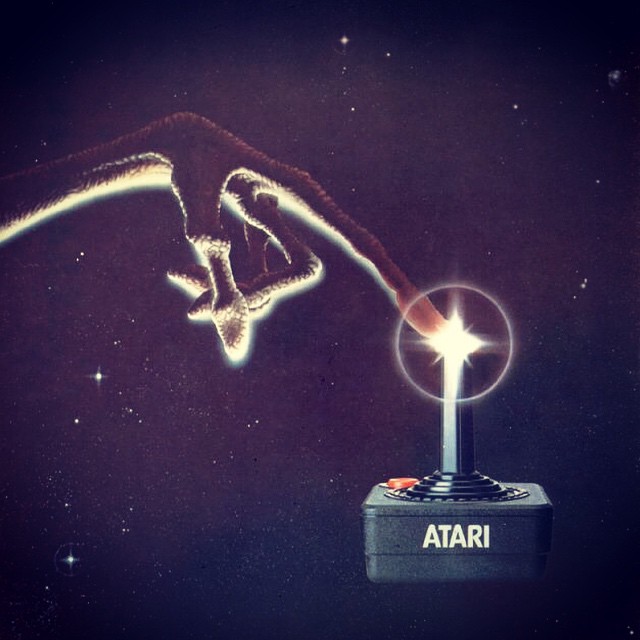This image is an advertisement for Atari, set against a mesmerizing outer space backdrop. The background transitions from a deep blue at the corners to a rich purplish hue towards the center, dotted with sparkling stars. Dominating the left side of the image is E.T.'s iconic illuminated finger, reaching out to touch the tip of an Atari joystick. The fingertip and the joystick create a focal point with a glowing white circle emphasizing their connection. The joystick itself extends down to a sleek black box, adorned with concentric rings and featuring a prominent red button. The front of the black box proudly displays the iconic ATARI logo in bold, white capital letters, completing the striking visual presentation.